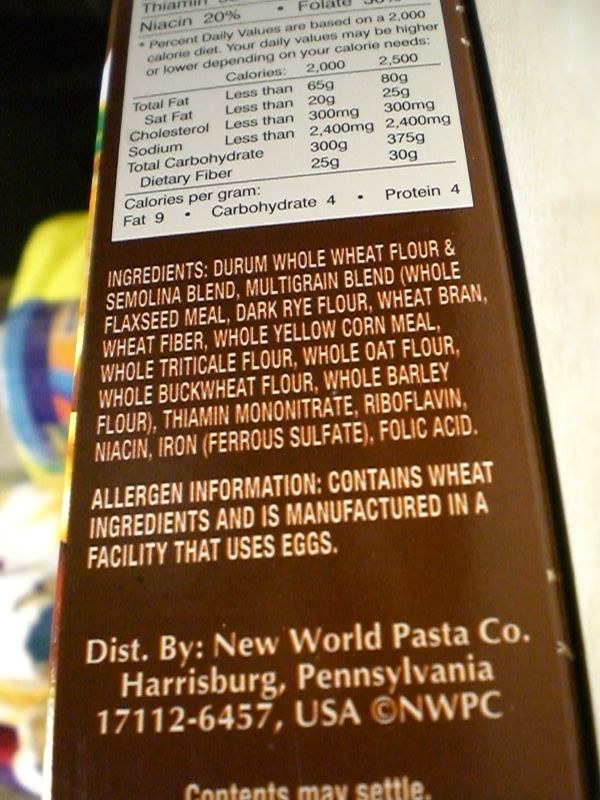The image displays the side of a brown pasta box featuring a partial nutritional label and a comprehensive ingredient list. The nutritional information, presented in a white and black square format, is only partially visible and mentions daily values based on a 2,000-calorie diet, with categories like total fat, saturated fat, cholesterol, sodium, and carbohydrates. The ingredients, written in a white to cream color typeface, include durum whole wheat flour, semolina blend, whole flaxseed meal, dark rye flour, wheat bran, wheat fiber, whole yellow cornmeal, whole triticale flour, whole oat flour, whole buckwheat flour, whole barley flour, thiamin, mononitrate, riboflavin, niacin, iron, and folic acid. Additionally, the allergen information indicates the presence of wheat and notes that the product is manufactured in a facility that uses eggs. Distributed by New World Pasta Corporation, located in Harrisburg, Pennsylvania, 17112-6457, USA, the box also states copyright NWPC and mentions that contents may settle.